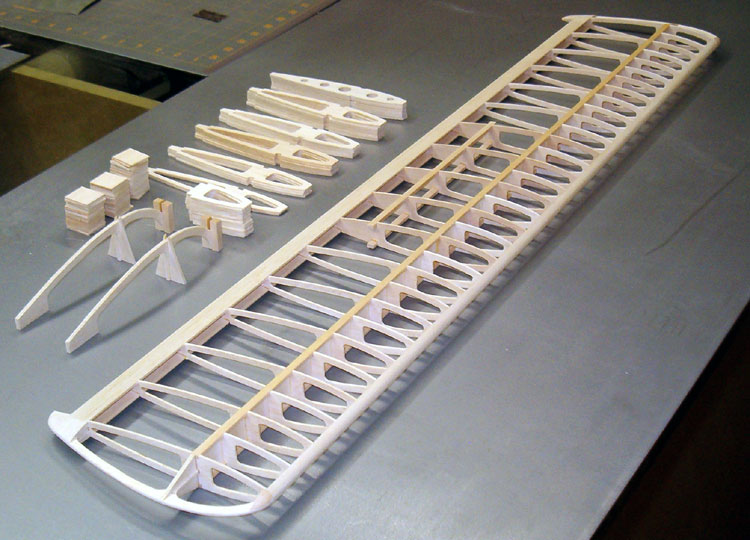The rectangular image depicts a partially assembled model airplane wing, displayed on a gray metal workbench with grid markings. The wing's framework, likely crafted from softwood such as balsa or basswood, features a detailed latticework pattern. This framework includes oval-shaped pieces with central connectors, suggesting intricate truss construction. Several smaller wooden components, including square blocks and elongated strips, are organized next to the main structure. These elements rest on a textured metal counter, which extends across most of the photo. Underneath the counter, a yellow bin and a wooden crate are partially visible. The overall scene suggests a meticulous assembly process of a hobbyist-grade airplane model.